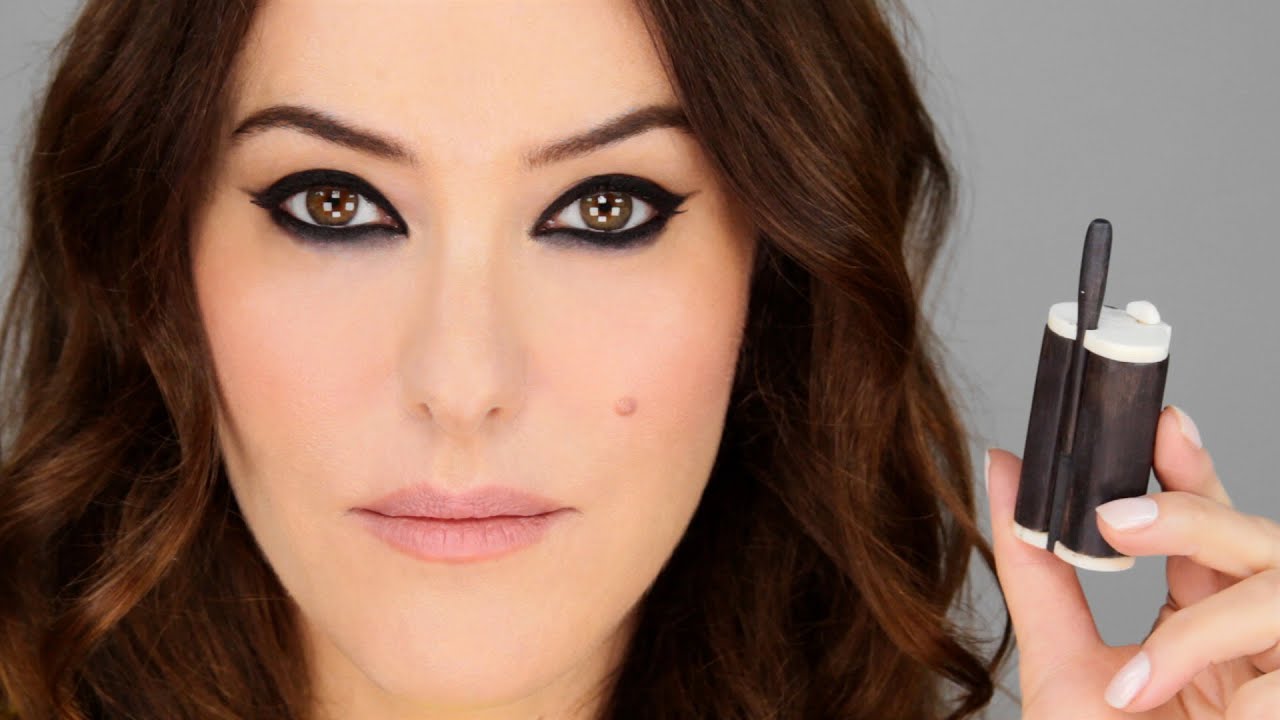In this color landscape-oriented photograph, a woman with striking brown eyes heavily highlighted with mascara, eyeliner, and eyeshadow gazes up at the viewer. Her brown, shiny, wavy hair frames her face, which is adorned with a noticeable pimple and medium-sized lips coated in pink lip gloss. She holds a small, black cylindrical device with white edges and a thin black brush on the right side of the image, near her cheek but not touching it; this is likely an applicator for eyeshadow, suggesting a makeup product advertisement. Her hand with white fingernails is prominently visible. Reflections of four screens in the shape of a T are visible in her eyes, adding a modern touch. The background is mostly white, further highlighting her facial features and the product she showcases. The detailed realism of the photograph gives it a highly representational style.